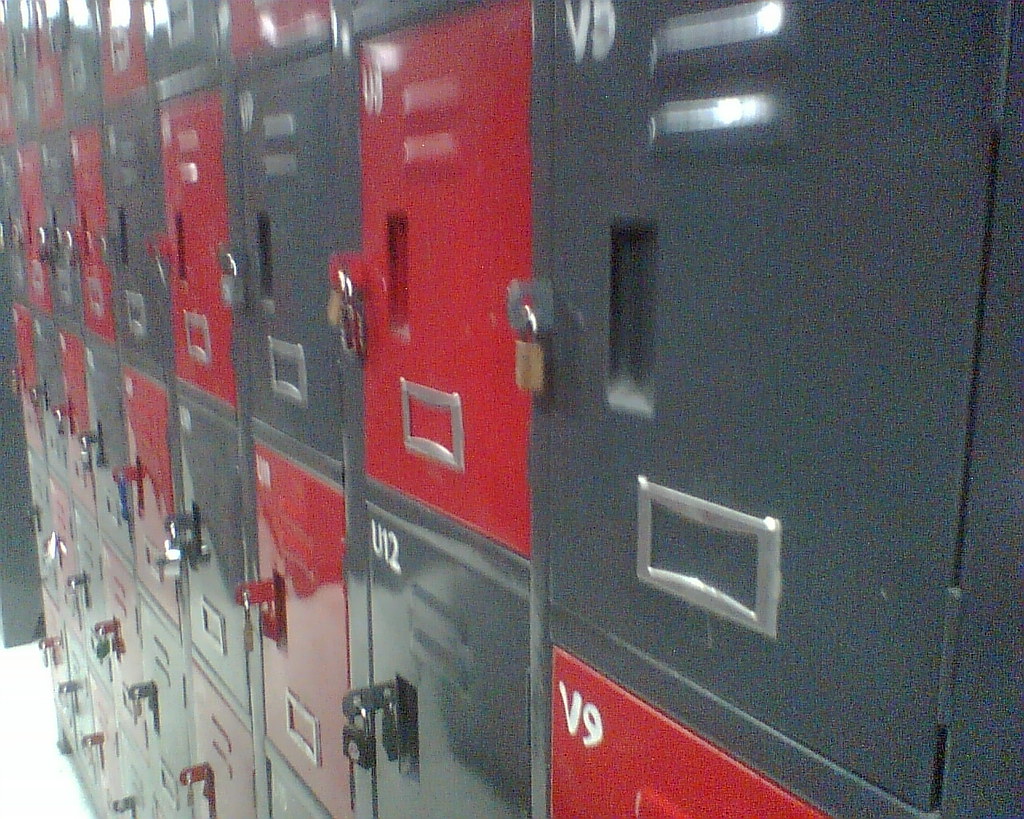The photograph depicts a vibrant locker room setting, likely situated in a non-traditional venue such as a gym or local storage facility, distinguished by its small cubby-sized lockers. The arrangement features alternating gray and red lockers, each securely fastened with either gray or golden locks that appear to require keys. The lockers are systematically labeled with a combination of letters and numbers, such as "U12," "U11," and "V9," where it seems the letter changes with the row and the number with the column. The floor is white, though largely obscured by the lockers. Each locker also includes a middle slot designed to hold cards for names or additional identification. The overall color scheme presents a striking contrast of gray and red, with silver tags visible on the lockers, contributing to a visually organized yet vibrant atmosphere.